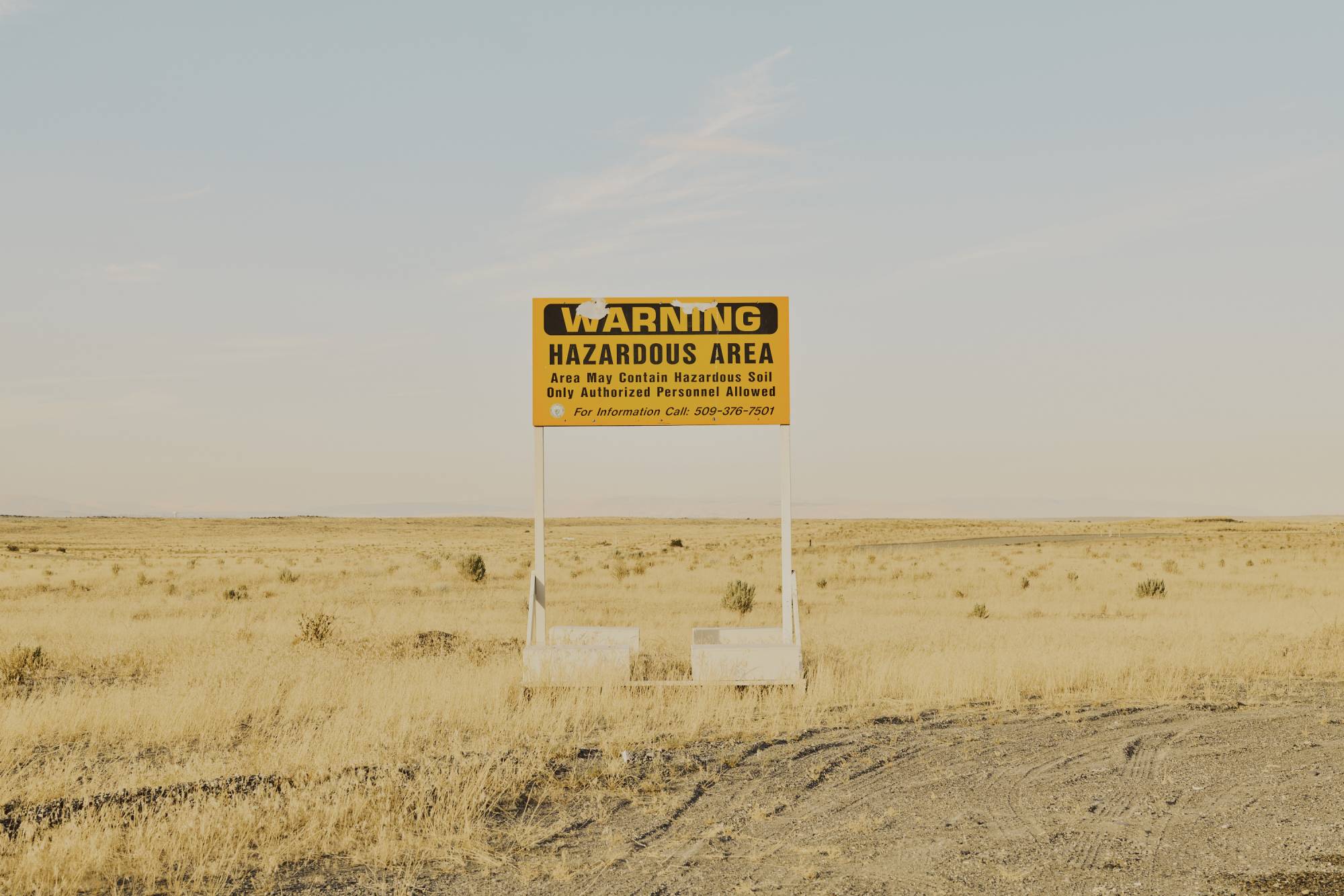The rectangular photograph captures a barren, flat field, dominated by a warning sign centrally placed on a white frame with two poles supporting a large rectangular yellow sign with black text reading: "WARNING HAZARDOUS AREA. Area may contain hazardous soil. Only authorized personnel allowed. For information call 509-376-7501." The foreground features a dirt path with multiple tire tracks positioned in the bottom right corner. The landscape behind the sign is an expansive meadow of short yellow grasses and sparse small green shrubs, devoid of buildings or mountains. The sky, occupying roughly half the image, is a light blue with thin, wispy clouds, suggesting an afternoon setting. The overall scene conveys a sense of desolation, with the field appearing largely lifeless and the sky casting a soft, late-day light.